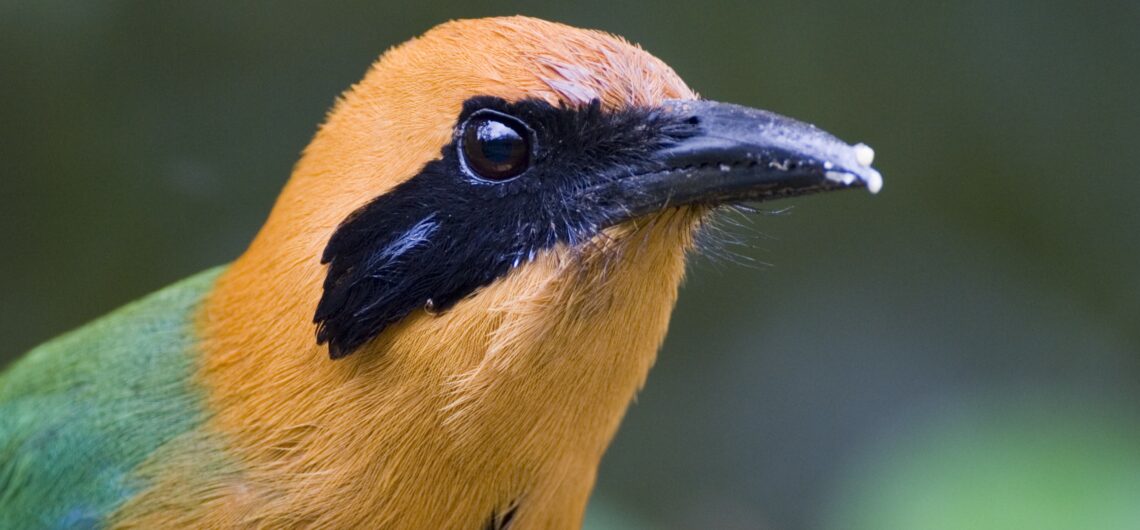This is a wide-angle, close-up photograph of a brightly colored bird, predominantly capturing its head and a portion of its neck and upper breast. The bird faces right, showing mainly the right side of its head and face at a three-quarter angle, so its rounded, orange-feathered head is prominently featured. The orange feathers extend from the top of its head down to its breast area. The bird also has a striking black beak, which is tipped with a white substance possibly indicating recent feeding. This beak continues into a black feathered mask that covers its cheeks and surrounds its black eyes, similar to the mask seen in cardinals, but extending slightly past the eyes and down the head.

The back of the bird's neck transitions into vivid green feathers, which continue down to its back. The image background is a blurred blend of deep greens with some areas of blue-green and bright green, creating a depth of field that keeps the bird's vivid colors and details as the main focus. The photograph is in a horizontal rectangle orientation and appears to have been taken with a wide-aperture lens, which enhances the clarity and focus on the bird while beautifully blurring the background. There is no text in the image.